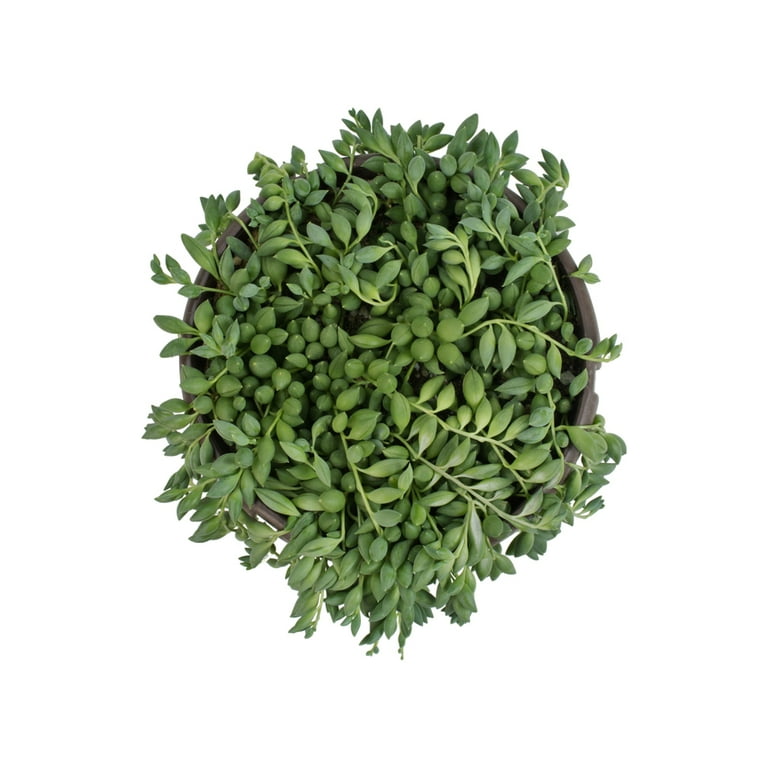This image features a lush, green plant overflowing from a brown pot, captured from an overhead perspective against a stark white background, suggesting a professional studio setting. The plant, potentially a succulent, has numerous stems densely packed with small, almond-shaped leaves and several tiny green bulbs or pods, which may be buds yet to bloom. The overall composition is dominated by the vibrant green of the foliage, with the brown rim of the pot just barely visible. The intricate network of leaves and bulbs nearly obscures the pot entirely, emphasizing the plant's fullness and vibrant health.